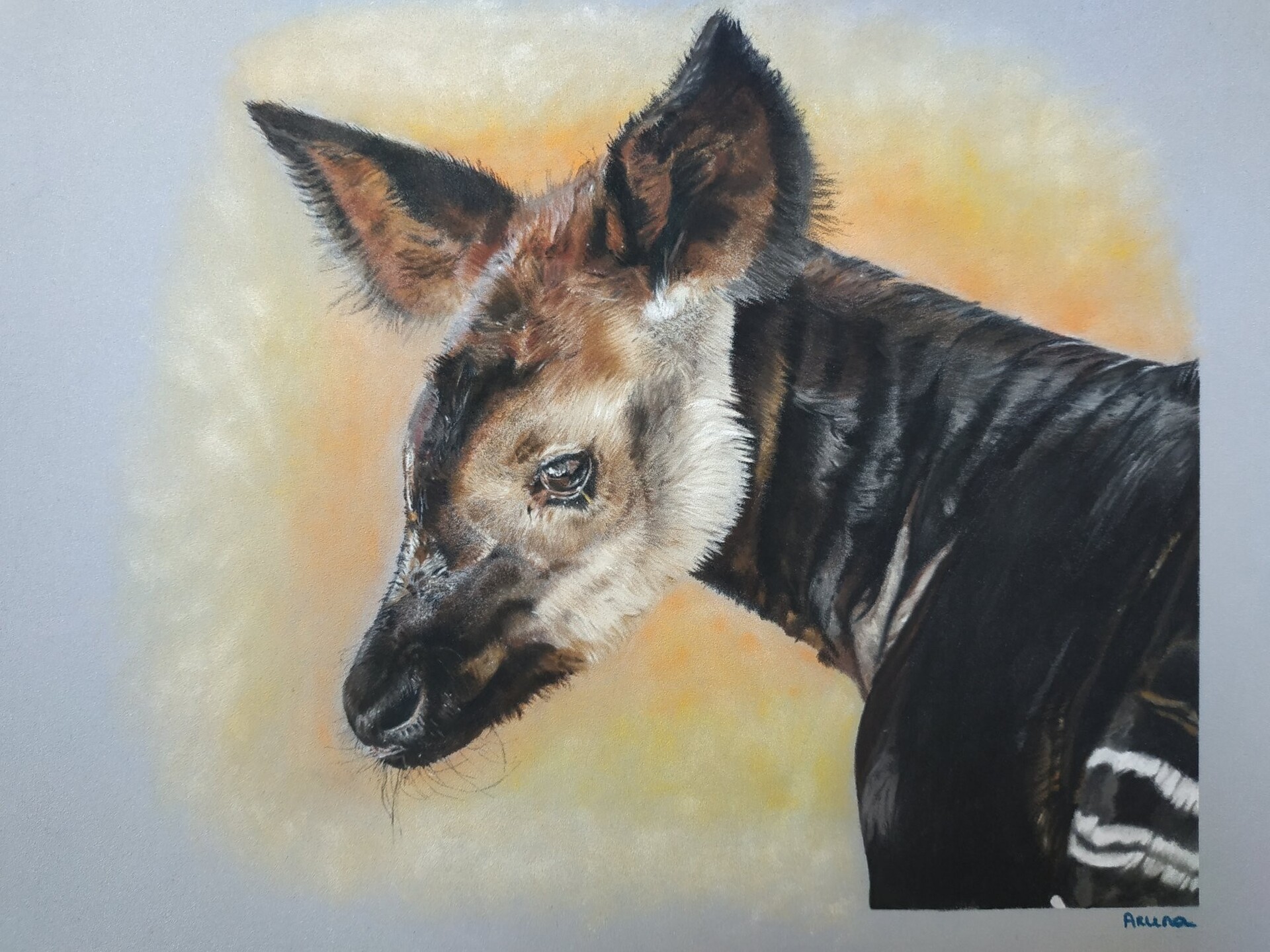In this oil painting by an artist whose signature appears to be "Aruna" in the bottom right, the background is predominantly a grayish color with a fuzzy circular pattern of light yellow to orange, creating a distinct contrast against the featured animal. The focal point is a unique creature that seems to be an imaginative hybrid of a wild dog, fox, jackal, and perhaps a hint of a zebra. The animal is depicted in a side profile facing left, showcasing a blend of intriguing features. It has pointy ears that are black on the outer edges and brown on the inside, along with a black nose featuring a large oval nostril. The animal's face exhibits a mix of light brown to light gray fur under and around the eyes, leading into a black and brown patterned forehead. The neck of the creature is adorned with black fur, resembling the ridges of a sweater, and extends into shoulders that alternate between black and black-and-white stripes interspersed with golden hues. With its black eyes and short hairs that echo the texture of a dog's coat, this fantastical animal captures a fascinating amalgam of characteristics, firmly placing the viewer's focus on its enigmatic presence against the contrasting pastel background.